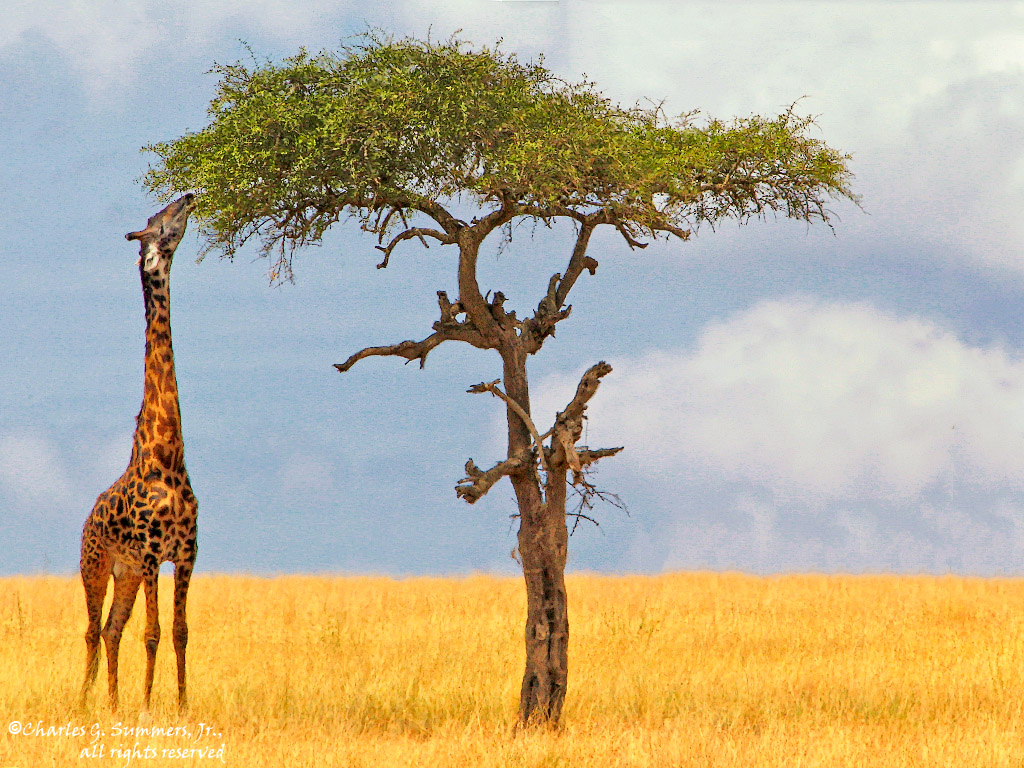This vivid photo captures an African savanna with a distinctive yellow grassy plain and a striking blue, albeit cloudy, sky. Dominating the center is a unique tree with thick, winding branches mostly barren except for a cluster of green leaves at the very top. To the left of the tree stands an elegant giraffe with an exceptionally long neck, small ears, and slender legs, its orange coat adorned with brown spots. The giraffe is reaching up, chewing the leaves from the sparse tree's highest branches. Subtle details, like possible small animals perched on the tree's branches, add depth to the scene. In the lower-left corner, a copyright notice reads: “© Charles G. Summers Jr. All rights reserved.”